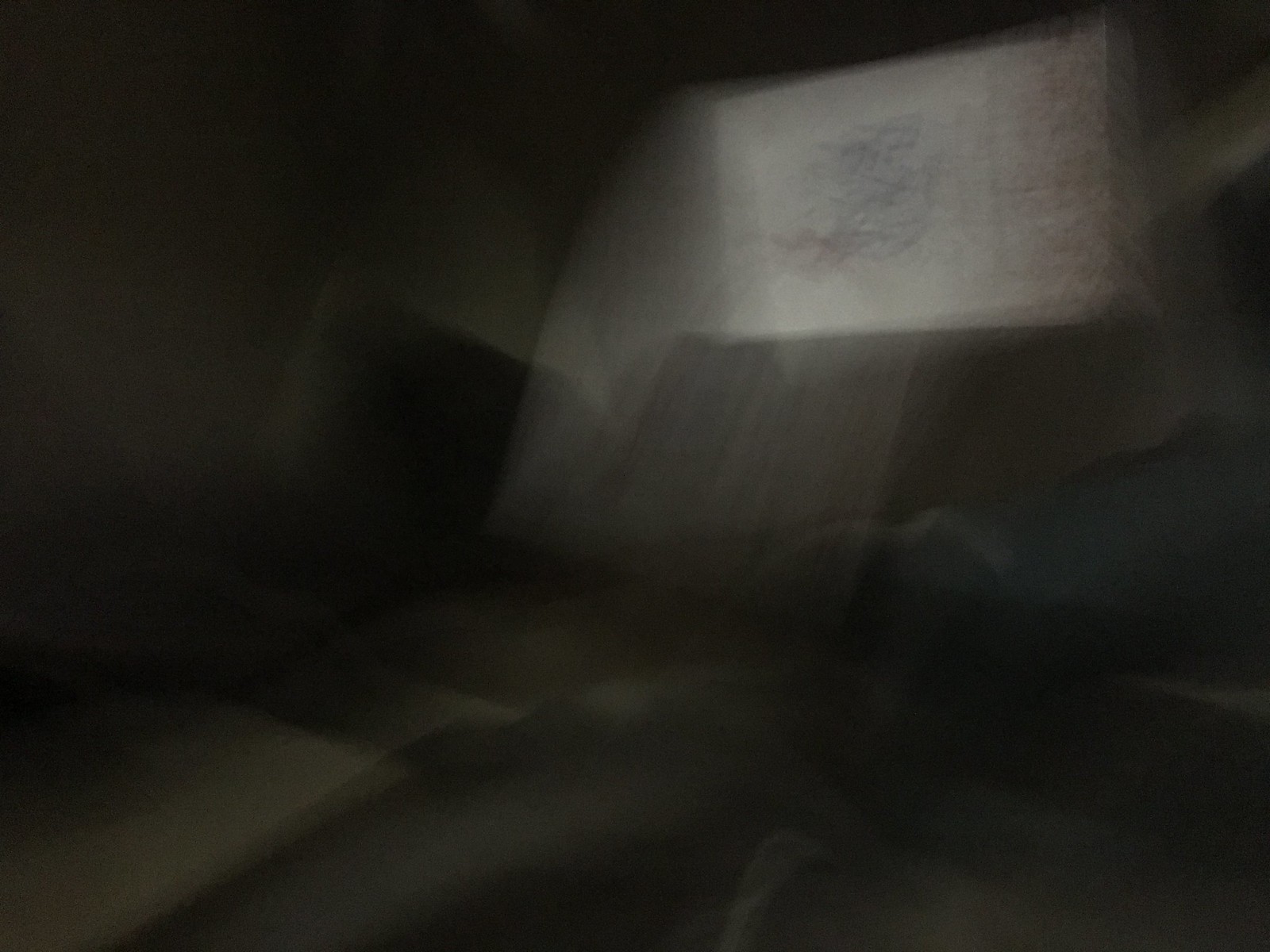The image is a black and white, heavily blurred photograph, which may intentionally appear abstract. The overall scene suggests an interior space that could be a bedroom or living room. Dominating the central portion is a large, dark recliner with a tall backrest. On the right side, there seems to be a bed occupying much of the space. Light filters through a window, creating a rectangular, bright reflection on the wall, hinting that the curtains might be partially closed, thereby diffusing much of the natural light. In the top right corner, there's an indistinguishable object that could either be a monitor, a screen, or perhaps a whiteboard with faint lines or data, accompanied by streaks of light that suggest movement or fog. The left-hand side blends organic and square shapes, possibly indicating other pieces of furniture or shadowy elements, contributing to the overall foggy and dreamlike atmosphere of the photograph.